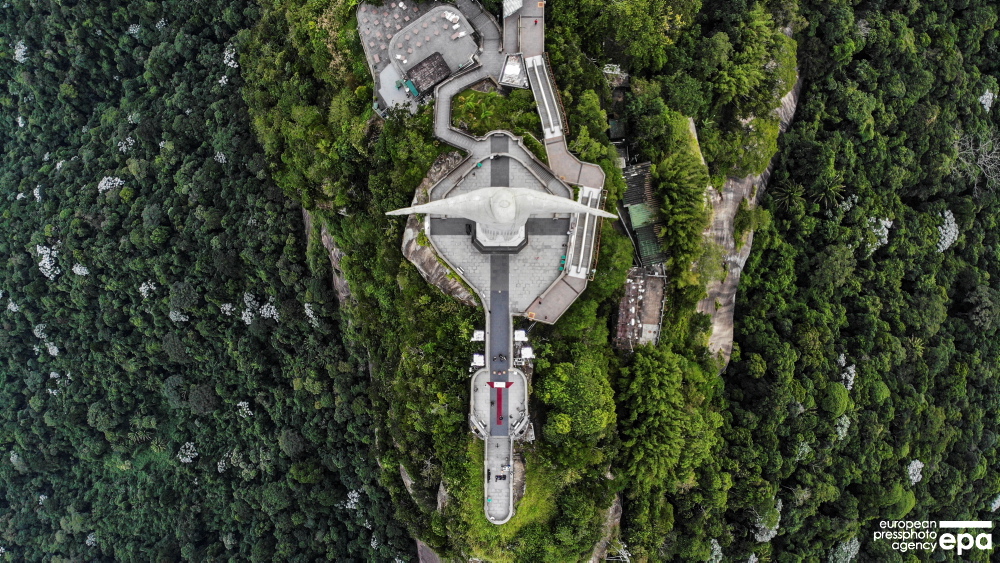This is an aerial view taken from a drone, showcasing the iconic Christ the Redeemer statue in Rio de Janeiro, Brazil. The statue, centrally positioned in the image, gives the appearance of a long, gray structure with a circular, halo-like portion at the top, reminiscent of a spaceship or a pistol in shape. Positioned almost vertically, with the front of the statue facing the bottom of the image, there are distinct pathways surrounding it, including a platform that overhangs the edge of the mountain, from which tourists can be seen observing the stunning panorama. The landscape around the statue is dominated by dense greenery, encompassing a hillside or mountainside rich with trees and various flora. The bright sunlight illuminates the right side of the terrain, while areas of shadow define the left. Additional buildings can be seen dispersed amongst the forested area. A small note in the bottom right corner credits the European Press Photo Agency (EPA) for this breathtaking capture.